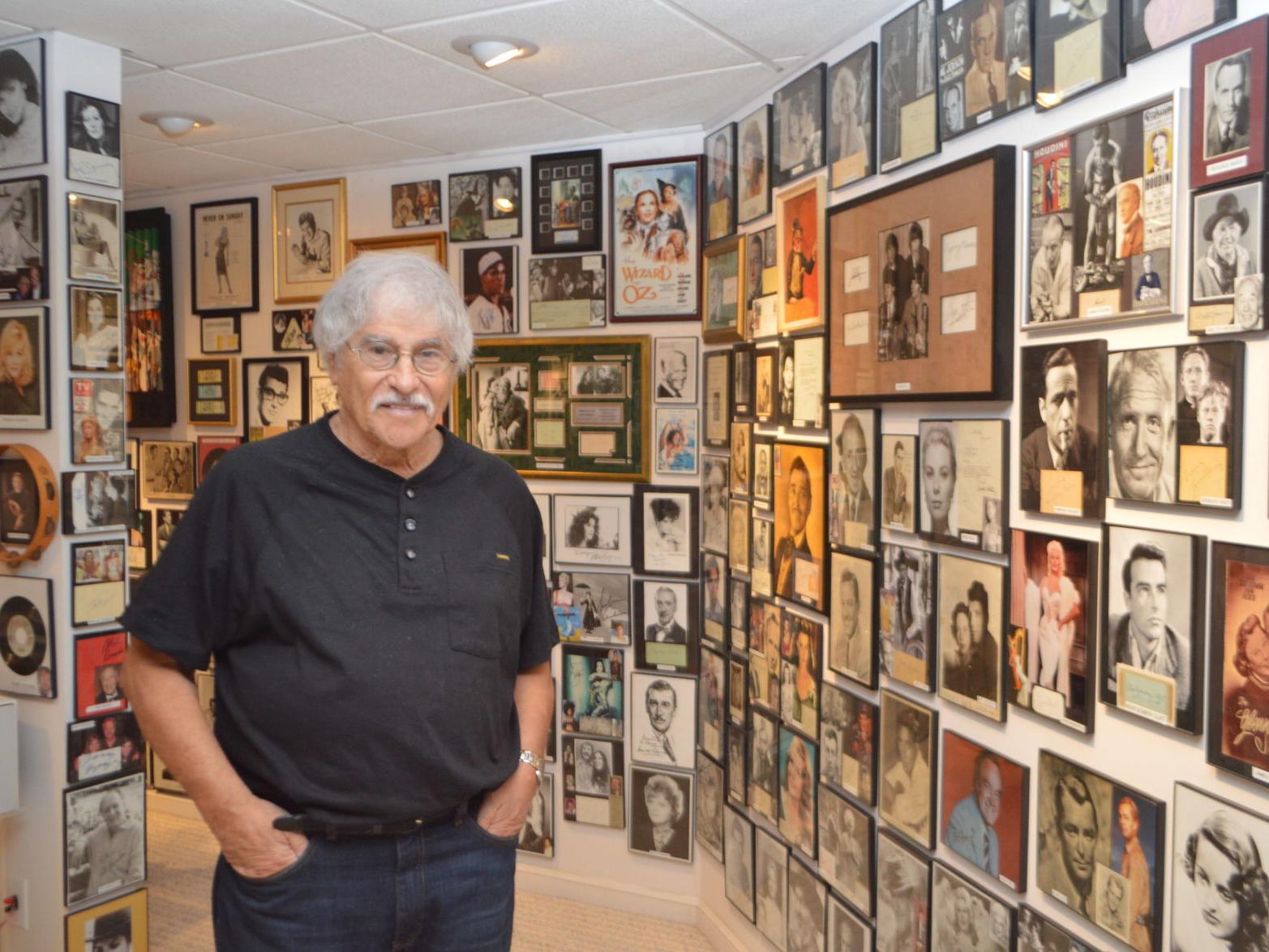The photo features an elderly gentleman with gray hair, a gray mustache, and glasses, standing in a memorabilia-filled room or hallway. He is dressed in a black t-shirt and dark blue jeans. The walls behind him are adorned from floor to ceiling with framed photos, portraits, and movie posters of classic film stars from the early 1920s to the 1950s, with some pieces extending into the 1960s. Each framed piece often includes a signature below the image. Some photos are in color, while others are in black and white, and the collection appears extensive, featuring over a hundred individual items. Notable among the collection is a poster for "The Wizard of Oz." The setting suggests it could be a personal collection or a shop, likely belonging to the man in the photo.